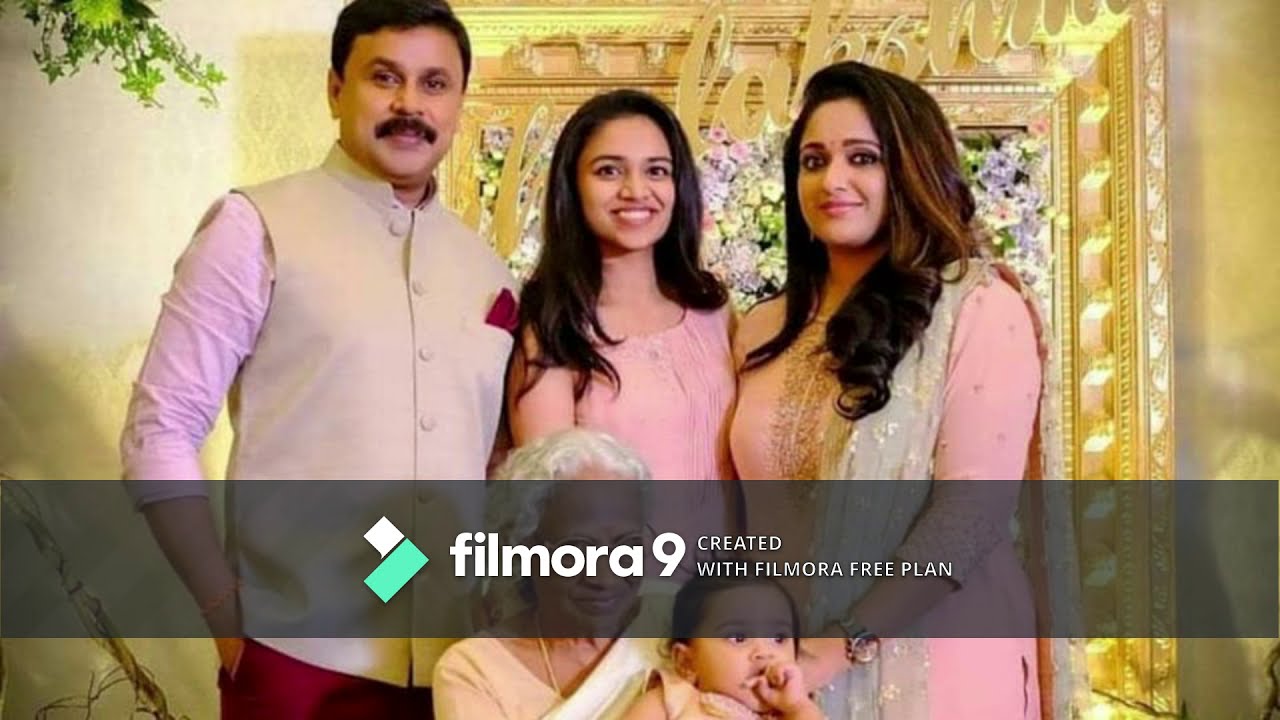This detailed, wide rectangular photograph captures an Indian family standing against a light yellow wall adorned with yellow lace patterns. On the right side of the wall hangs a floral painting framed by an ornate, thick gold, yellow, and pink border with cursive golden text diagonally across it. The family comprises five members, displaying generational diversity. In the back row, starting from the left, is the father, a man with light tan skin, black hair, and a mustache, wearing a yellowish vest over a white or possibly pink shirt. To his right stands a younger girl, his daughter, with long black hair dressed in a pink tank top. Next to her, on the far right, is the mother, also with long black hair, dressed in a traditional pink Indian dress with a scarf. In the front row, an elderly woman with whitish hair sits while holding a baby. The family's expressions are warm and content, all smiling for the camera. Over the lower portion of the image, a partially opaque gray rectangle reads, "FILMORA 9, Created with Filmora Free Plan." To the left of this text is a small brand logo, consisting of a green rectangle next to a white square.